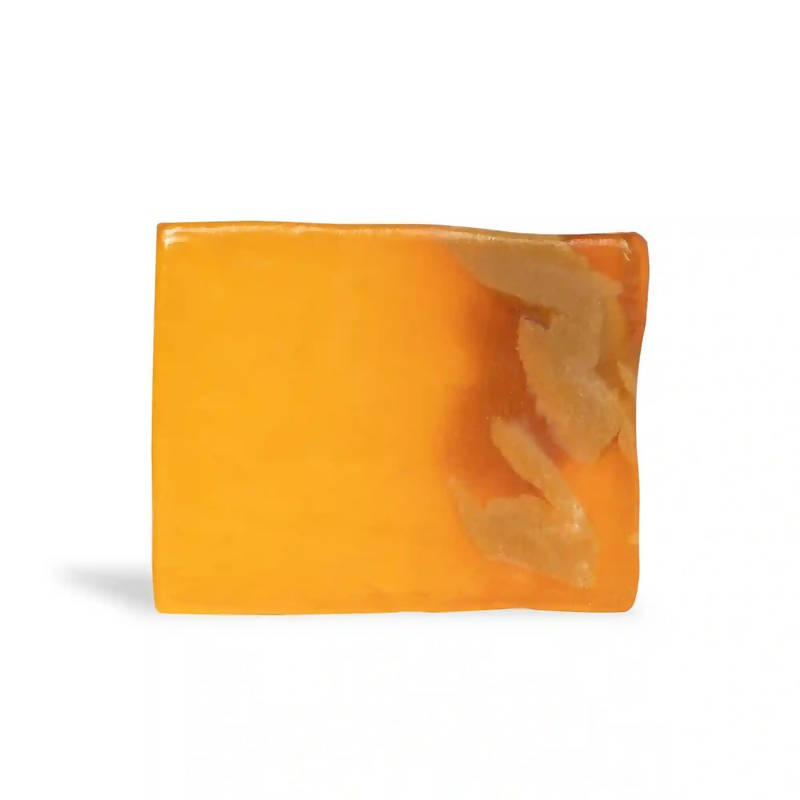This image features a square-shaped object with uneven edges, situated in the center of a plain white background. The object appears to be a piece of precious stone or possibly homemade or organic soap. Measuring approximately a quarter of an inch in thickness, its colors transition from light orange on the left to a deeper orange, and then to a red-orange hue before tapering off again on the far right. The surface displays varying shades of orange and gray shapes, primarily on the right side, which appear naturally embellished rather than man-made. Its texture looks somewhat jelly-like, with portions resembling yellow gel or honey gold, giving a translucent quality. Overall, the image captures the fine details and rich gradients of the square-shaped item against a stark white background.